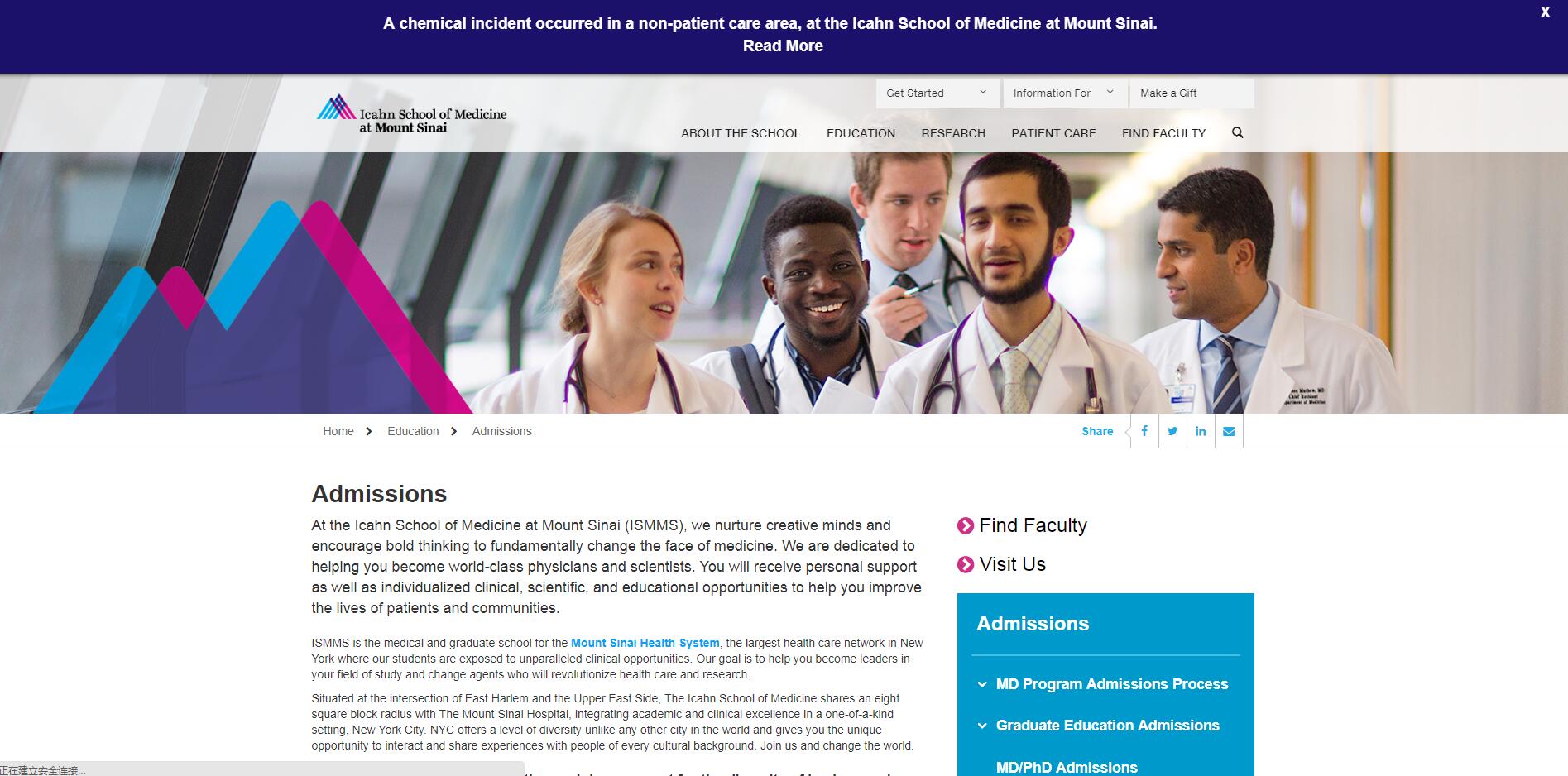The webpage belongs to the Ike Aiken School of Medicine at Mount Sinai, evidently a renowned medical institution. At the top of the page, there is a prominent blue bar with an urgent notification in white text announcing: "A chemical incident occurred in a non-patient care area at the Ike Aiken School of Medicine at Mount Sinai." A "Read More" link is provided for additional details.

Just below the blue bar is the school's distinctive logo, a triangle composed of three different colored lines, with the text "Ike Aiken School of Medicine at Mount Sinai" adjacent to it. The main navigation menu is situated next to the logo, featuring options such as About the School, Education, Research, Patient Care, and Find Faculty.

Above the navigation menu, there are three small search bars. It's challenging to discern their labels due to their tiny font, but they appear to offer options like "Get Started," an indeterminate second option, and "Make a Start" for the third.

The central content of the page features a large, attention-grabbing photograph that stretches across, roughly three times the height of the top blue bar. To the left of the image, the school’s logo is prominently displayed, albeit much larger than before. The photo depicts a diverse group of five individuals, all dressed in medical white coats. This group includes one female and four males of varying racial backgrounds, including White, Black, and possibly Indian. They appear engaged and cheerful, either interacting with each other or looking directly at the camera, all positioned in what seems to be a hospital hallway.

Beneath the photograph, there is a section dedicated to admissions information. It is labeled "Admissions" and contains three paragraphs, although the last two paragraphs are somewhat illegible. Alongside this section, there are links labeled "Find Faculty" and "Visit Us." Additionally, in the lower right corner of the page, there is a small blue rectangle offering more specific options such as Admissions, MD Program Admissions Process, and Graduate Education Admissions.

Overall, this webpage provides substantial information and navigation options for those interested in the Ike Aiken School of Medicine at Mount Sinai.